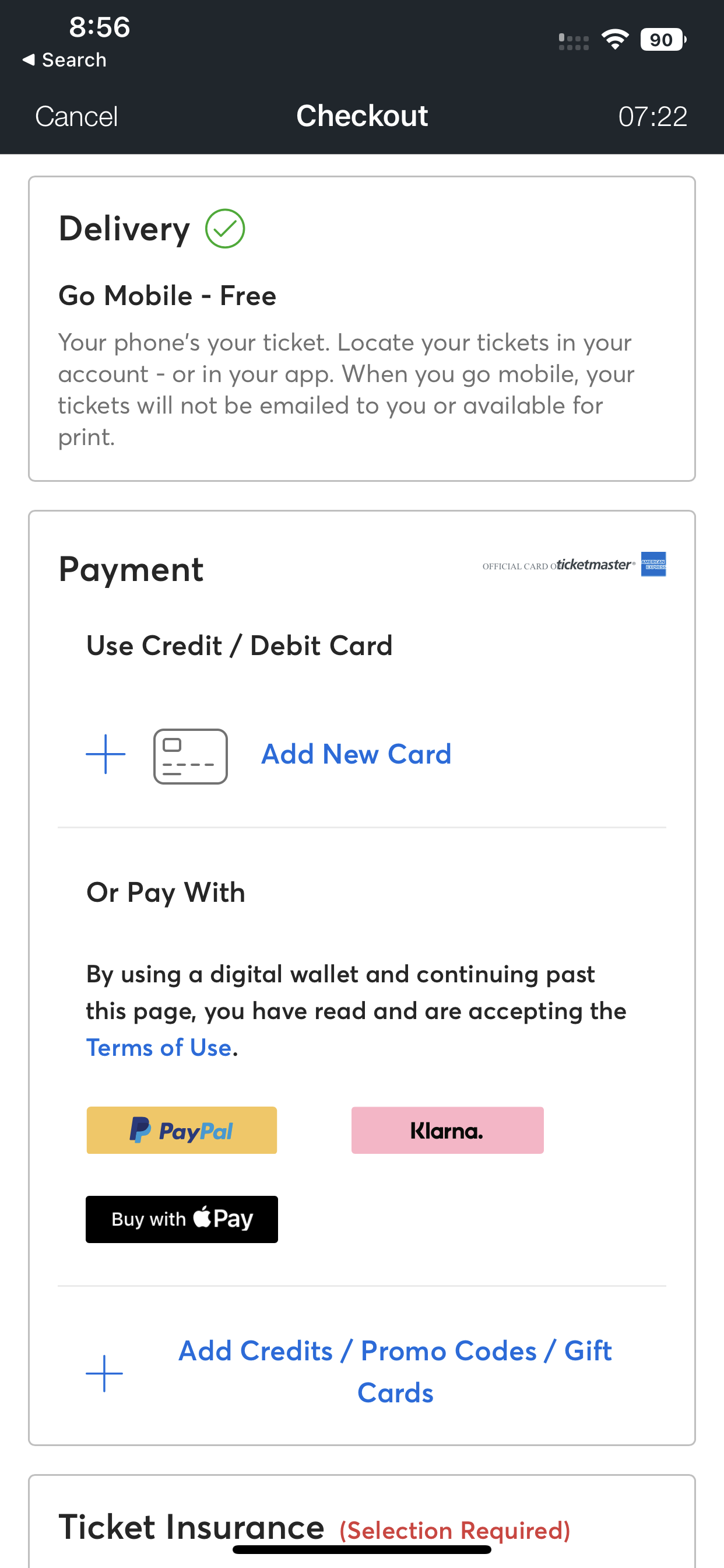An image showing a green user interface with a white background, focusing on the checkout screen numbered 722. The battery level is displayed at 90%. There are options to cancel and to choose delivery. The message encourages users to utilize mobile ticketing, advising that tickets can be found in their account or app, and specifying that mobile tickets will not be emailed or available for print.

The payment options include using a credit or debit card, adding a new card, or paying with a digital wallet. As users proceed, it is stated that they are agreeing to the terms of use, which is clickable and highlighted in blue. Payment methods featured include PayPal in a yellow rectangle, an option branded as “Klama” (possibly Klarna) in a pink rectangle, and Apple Pay represented by a black rectangle with an apple icon.

At the bottom, there are sections to add credit or promo codes, gift cards, and an option for ticket insurance, with a note in red indicating "selection required".